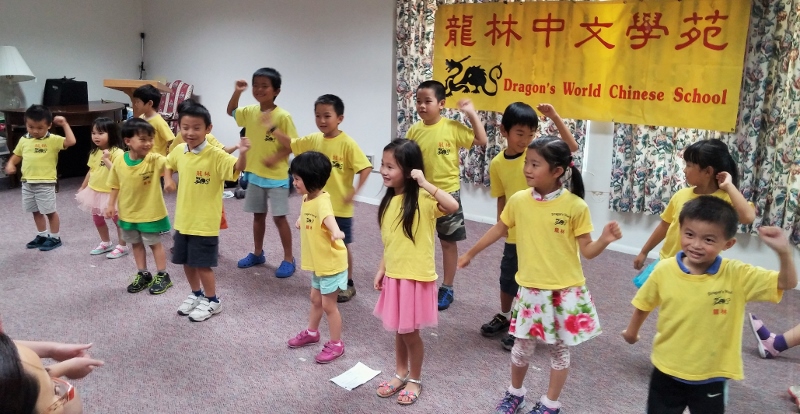The image depicts a lively scene of young children, likely between the ages of three to seven, performing or dancing at what appears to be a kindergarten or early primary school, named Dragon's World Chinese School. The children, who appear to be of Chinese descent with dark black hair, are all dressed in yellow t-shirts that match the prominent banner behind them. This large yellow banner, adorned with red Chinese text and an icon of a dragon, prominently displays the school's name in both Chinese and English. The performance takes place on a carpeted floor, likely indoors, with several pieces of furniture scattered around. In the bottom left corner, a woman with glasses, possibly a teacher or parent, observes the event. The background features two windows with floral curtains, adding to the cheerful atmosphere of the room. Overall, it is a colorful and dynamic scene capturing a moment of joy and cultural celebration among the children.